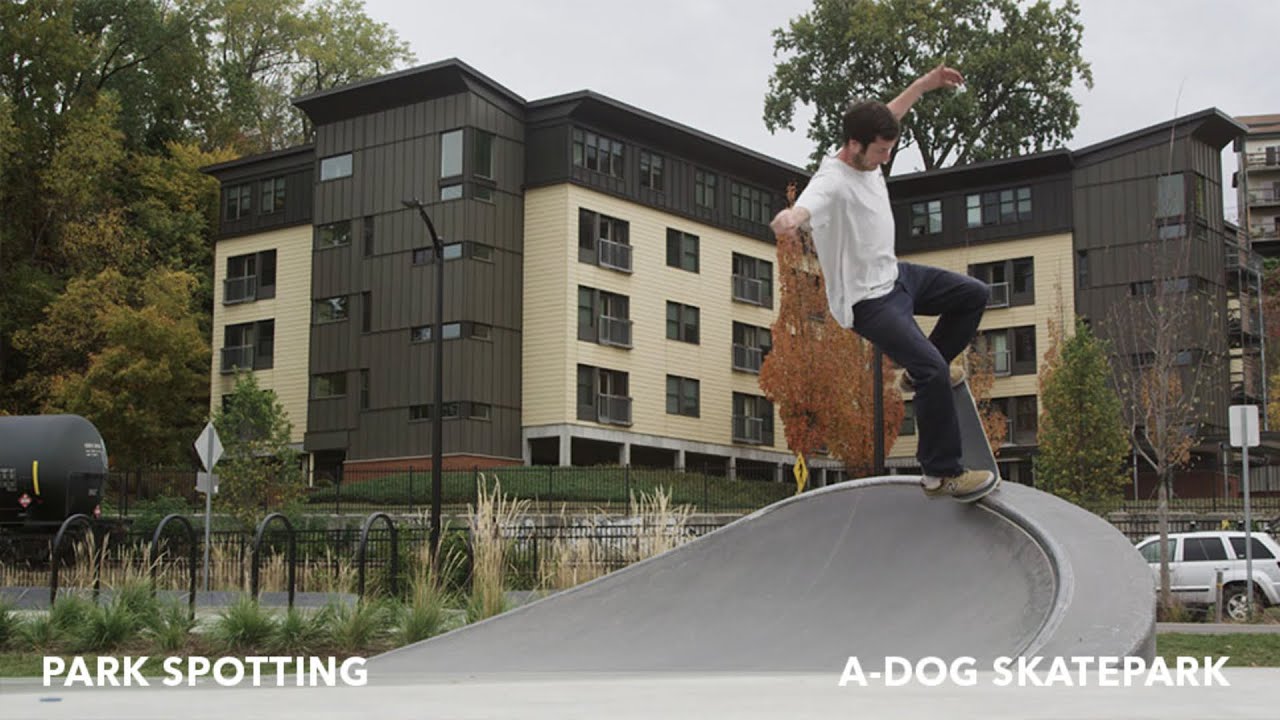The picture features a young Caucasian male with short brown hair, wearing a white t-shirt, dark pants—possibly black jeans—and tan shoes. He is skillfully riding a black skateboard along a thin, curvy concrete ledge in an outdoor skate park. This gray ledge starts from the left-hand side and slopes upward to form a ramp, on which he is performing a move with his arms stretched out to maintain balance. In the background, there's a large, multi-story building, which is tan and dark brown with numerous windows and balconies, resembling a modern apartment complex. A few cars, including a silver SUV and a tanker, are visible between the skate park and the building. The scene is set on a cloudy day with a grayish-white sky, and large trees and sidewalks frame the area. Along the bottom of the image, white text reads "Park Spotting" and "A Dog Skate Park."